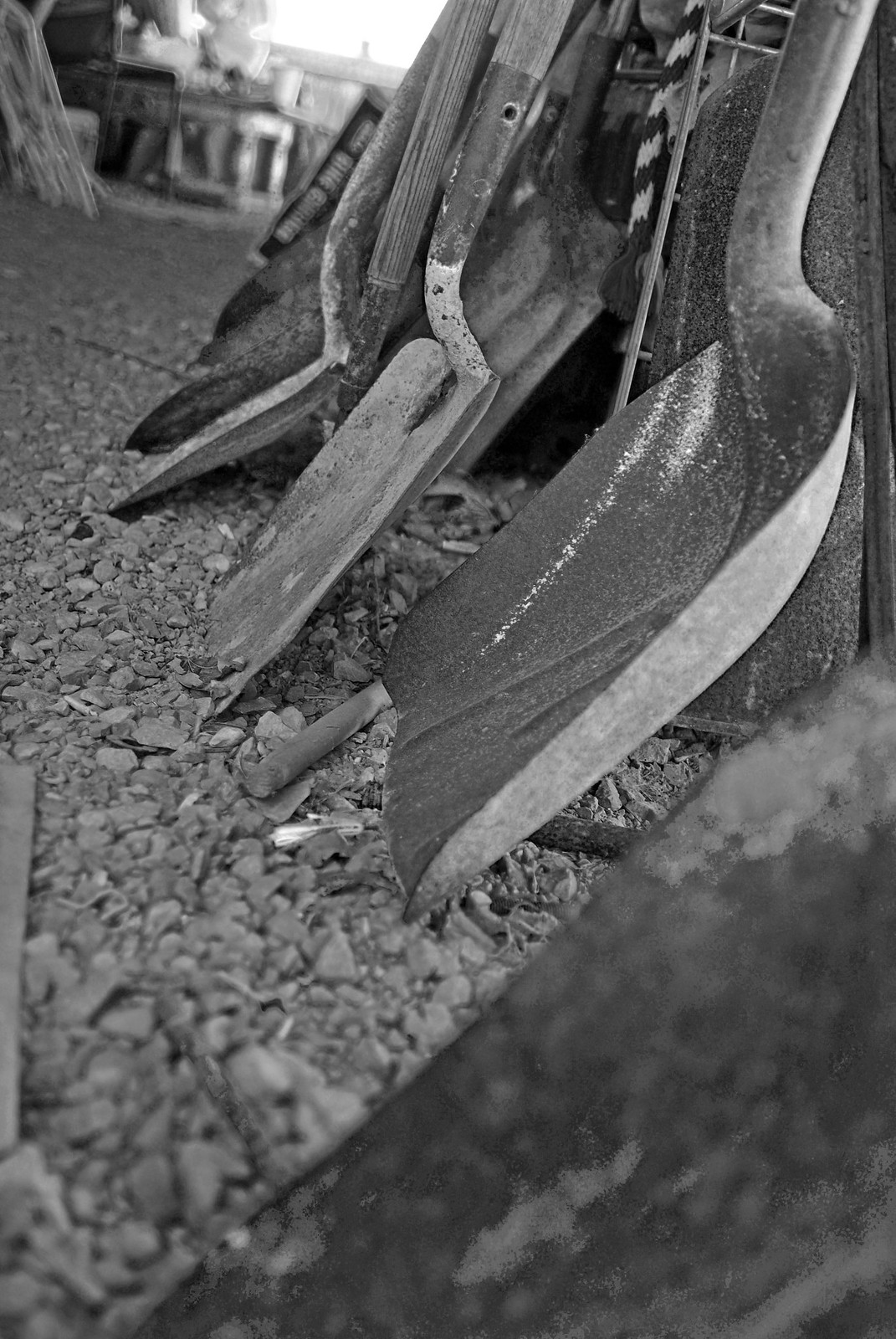This is a detailed black-and-white photograph of a rocky ground, which appears to be part of a tool shed or a similar setting. Dominating the foreground are several shovels, primarily metal with a mix of wood and metal handles. The shovels are arranged in a line, leaning against a concrete barrier. The image provides a clear focus on at least two to three shovels, while others appear more out of focus, suggesting a total of around six to seven shovels.

The ground is covered in numerous pebbles, small stones, and debris, adding to the gritty, construction-like feel of the scene. Among the debris are small wooden blocks and cylindrical objects scattered across the ground. The background is blurred, revealing hints of possible furniture, like chairs or a table, and some indistinct objects, including a bag that could contain mulch or fertilizer and a box with illegible, upside-down lettering. A cord with a swirling pattern is also visible between two of the most prominent shovels.

The lighting in the photograph is flat, enhancing the starkness of the black-and-white contrast. Despite the blurriness of the background elements, the image effectively captures the detailed texture of the shovels and rocky ground, making them the focal points of the scene.